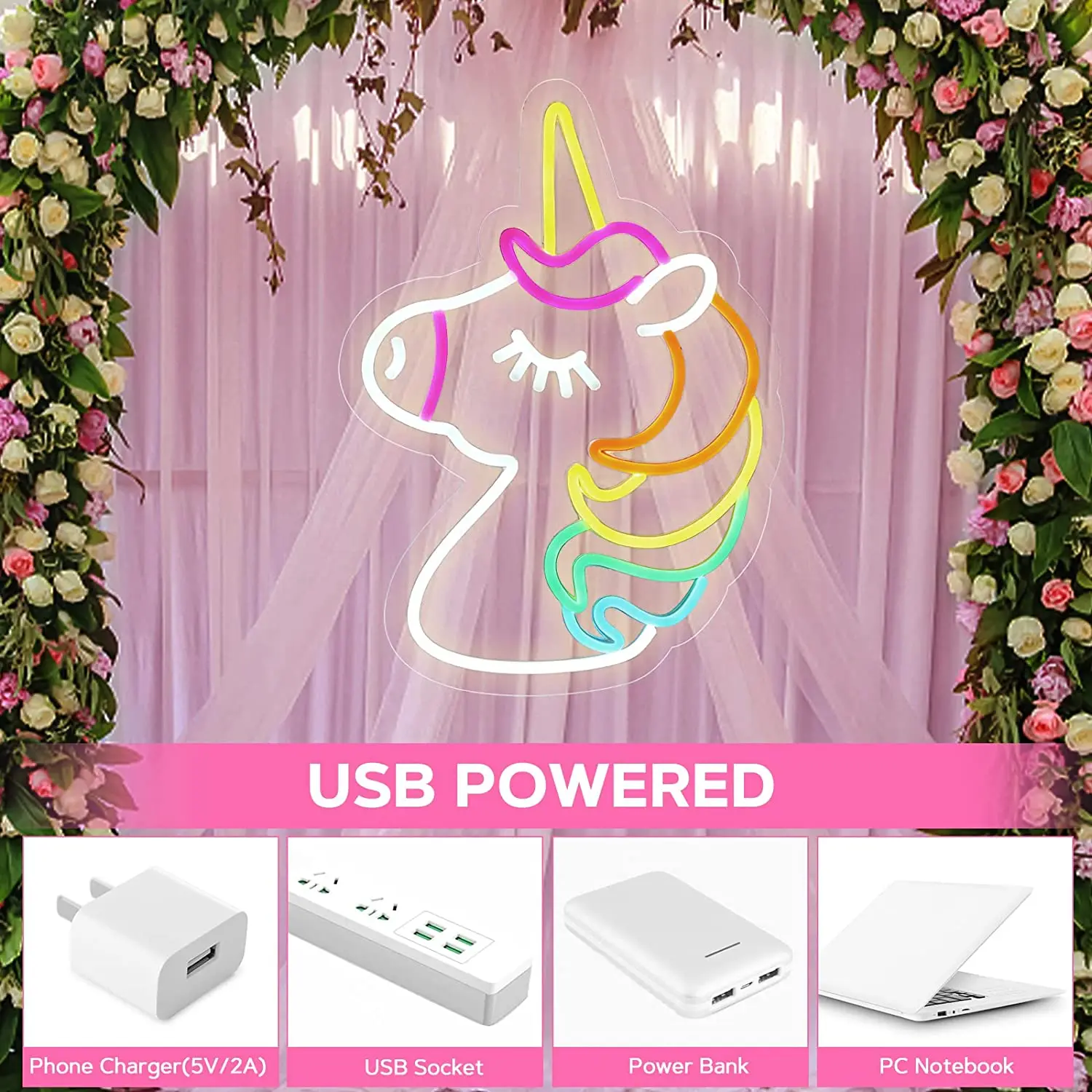This is a square-format advertisement featuring a combination of photography and illustration, showcasing various USB-powered devices. The background is adorned with an archway of pink, white, and light purple roses interspersed with greenery, framing the image from the top and sides. Hanging in the center is a white chiffon curtain, complemented by additional angled drapes. 

Front and center, a neon outline of a unicorn adds an eye-catching element. The unicorn's horn is yellow, its face is white with an eyelash, and its mane boasts a blend of pink, orange, yellow, blue, and green colors. Below this whimsical illustration, a pink horizontal rectangle with white text reads "USB powered."

At the bottom of the image, four white boxes display different USB-powered items against a white background. From left to right, these items include a phone charger labeled "5V 2A", a USB socket, a power bank, and a PC notebook. Each device is clearly featured with white text for easy identification. The advertisement combines photographic realism with stylized illustration to vividly highlight the products.